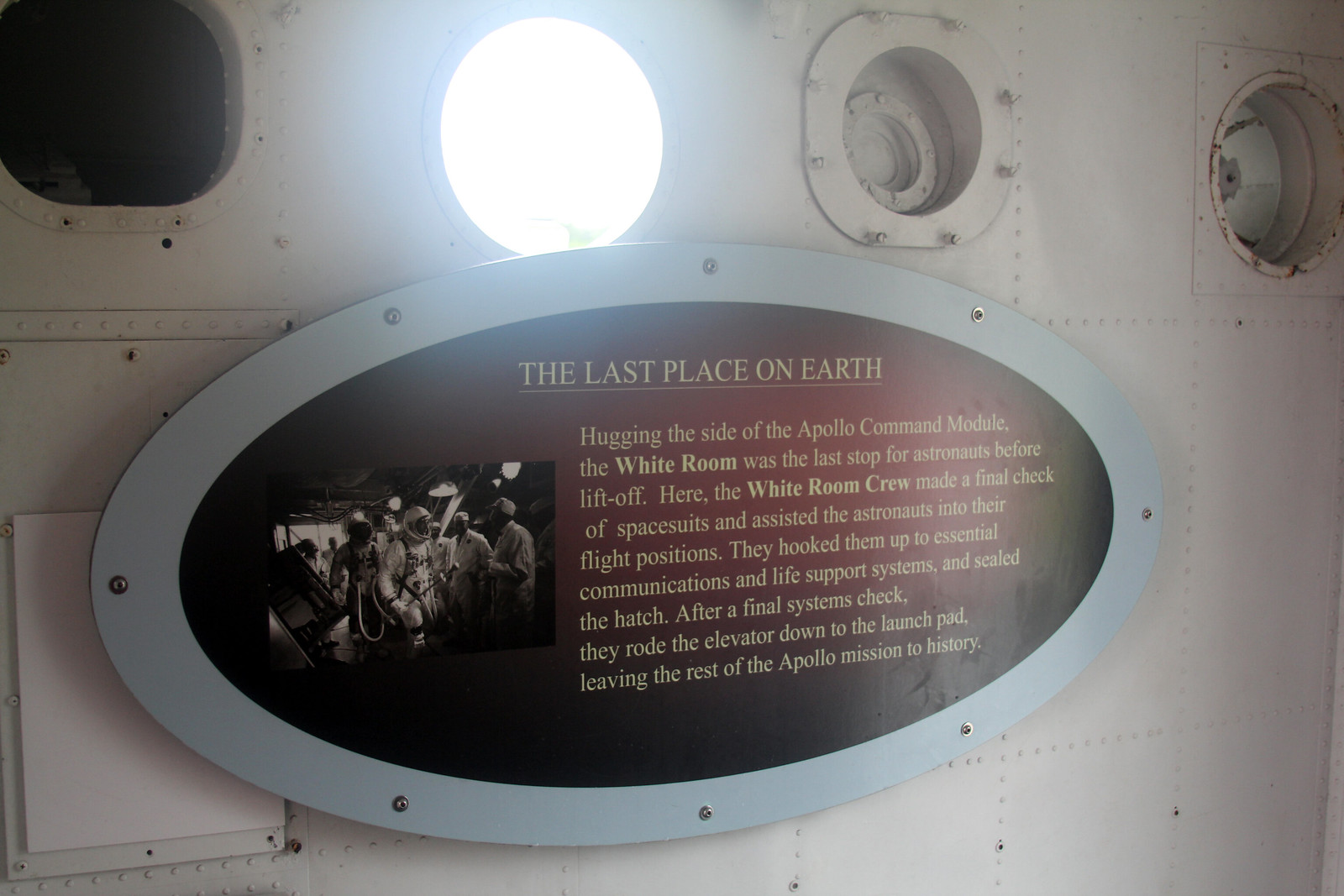This image captures a detailed historical marker titled "Last Place on Earth" located at a space launch facility, specifically attached to a wall reminiscent of a space shuttle's interior. The wall, probably part of a historical room used by NASA for astronauts' final preparations, is composed of hard white material, perhaps enamel, dotted with portholes and various valves. The ovular plaque itself has a white border with rivets securing it in place. The center of the plaque is red, featuring gold text and a black-and-white photograph on the left side depicting astronauts being assisted by the white room crew. The text reads: "Hugging the side of the Apollo command module, the White Room was the last stop for astronauts before liftoff. Here, the White Room crew made a final check of spacesuits and assisted the astronauts into their flight positions. They hooked them up to essential communications and life support systems and sealed the hatch. After a final systems check, they rode the elevator down to the launch pad, leaving the rest of the Apollo mission to history." The photograph highlights the crew and astronauts in their final moments before embarking on their mission, cementing the ‘White Room’ as a crucial element of space exploration history.